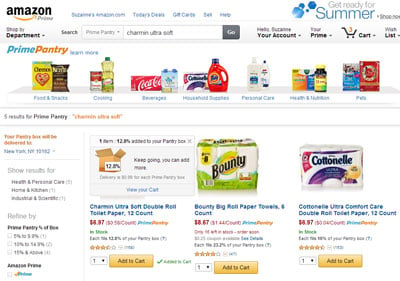Title: Amazon Prime Pantry Summer Promotions - June 2023

Description: This slightly blurry screenshot showcases Amazon Prime Pantry's summer promotions for Prime members. 

Details:
- **Welcome Section**: A cordial greeting to Suzanne from Amazon, indicating the user's account status. It also mentions three items in the cart and a wish list.
- **Prime Pantry Overview**: Highlights summer preparations with categories like food, snacks, cooking essentials, beverages, household supplies, personal care, health and nutrition, and pet products.
    - **Food & Snacks**: Images feature a bag of chips and a box of Cheerios.
    - **Cooking Essentials**: Displayed items include a Campbell's soup can and what appears to be a Crisco bottle of oil.
    - **Beverages**: Shown are a 12-pack of Coca-Cola and an indistinct multi-pack of bottled drinks.
    - **Household Supplies**: Highlighted products include Cottonelle toilet paper and Tide laundry detergent.
    - **Personal Care**: Features what seem to be Nivea and Eucerin products.
    - **Health and Nutrition**: Images include DayQuil, NyQuil, and a bottle of vitamins.
    - **Pet Supplies**: Appears to showcase Purina products and an unidentified item.
- **Prime Pantry Results**: Lists five key results for Prime Pantry, focusing on Charmin Ultra Soft, Bounty, and Cottonelle products.

The promotional message indicates these offers are perfect for getting ready for the summer season.